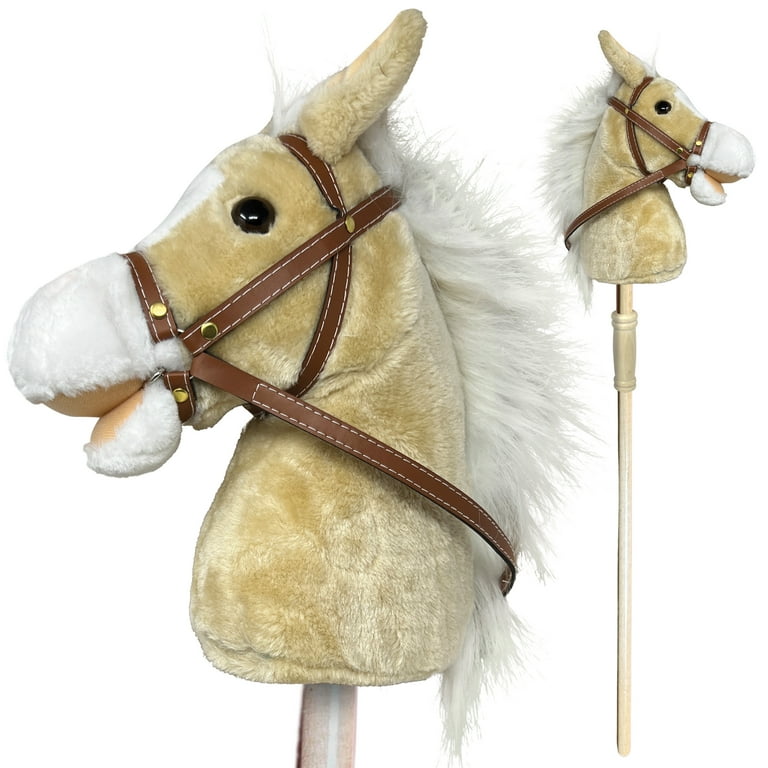The image is a color photograph in portrait orientation, focusing on a hobby horse toy, commonly known as a stick horse, designed for children. The horse head, which is the main subject, is crafted from a brown and white plush fabric with a white fuzzy mane. It features large stitched black eyes and a brown leather halter adorning its face. A distinct white stripe runs down its forehead and there is a white area around its mouth.

The horse head is mounted on a tall, cream-colored wooden pole with visible grain, which includes a thicker handle section marked by two bands at the top and one at the bottom. On the left side of the image, there's a close-up of the horse's head in profile, showing the nose pointing left and the mane flowing to the right. The ears stand upright, adding to the realistic appearance of the toy.

On the right side of the image, a more distant shot reveals the full length of the hobby horse, showcasing the entire stick. The image is set against a plain white background, emphasizing the toy without any distractions. This photographic composition highlights the intricate details and craftsmanship of the hobby horse, embodying a style of representational realism typical of product photography.